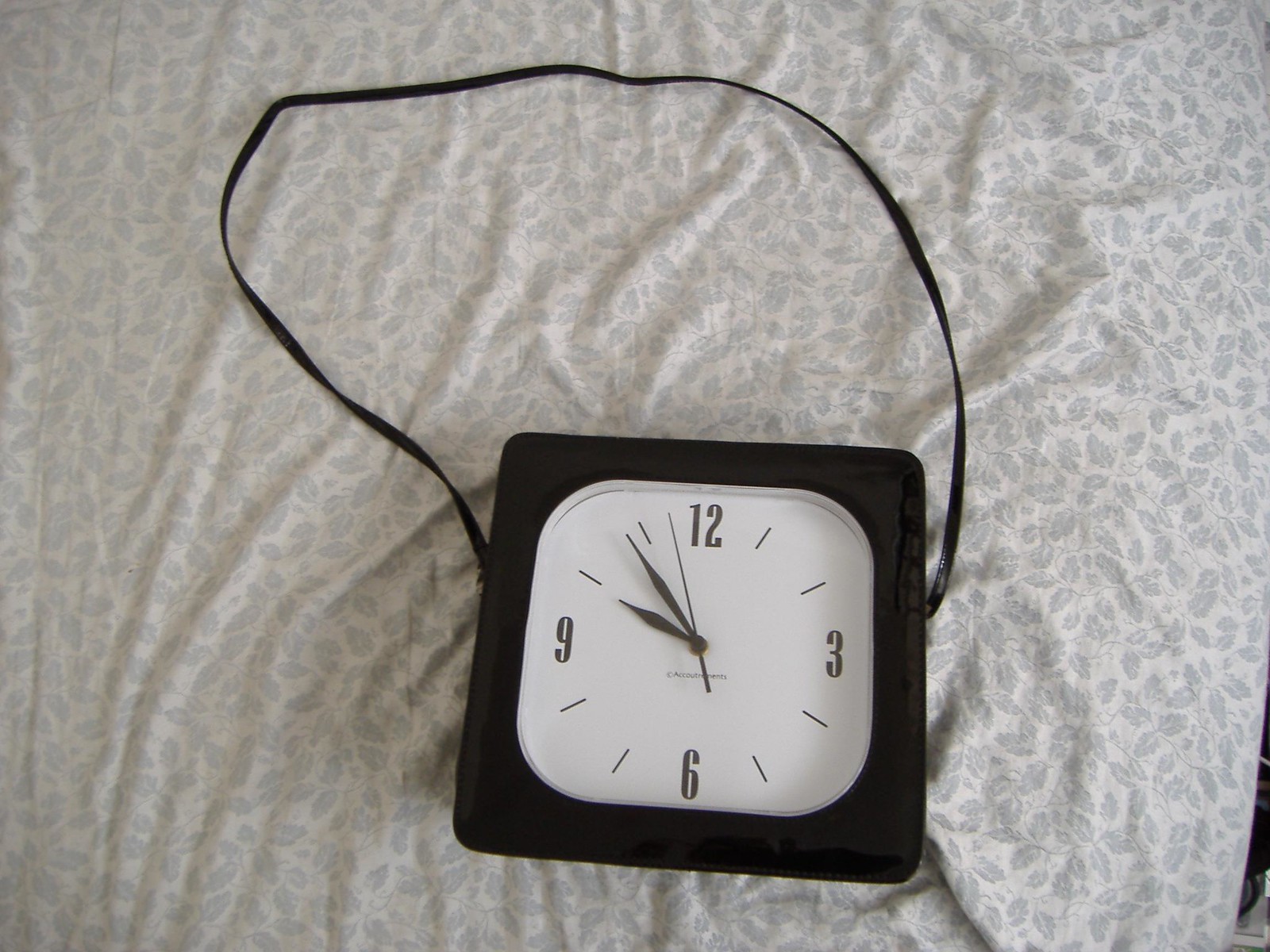A black faux leather purse in the shape of a square with rounded corners is positioned on a rumpled white bed sheet adorned with a lavender leaf design. The purse features a design resembling a clock face, complete with black numerals and black hour, minute, and second hands against a white background. The long, slender black strap of the purse extends across the bed sheet, giving the impression that the purse has been casually tossed onto the bed.